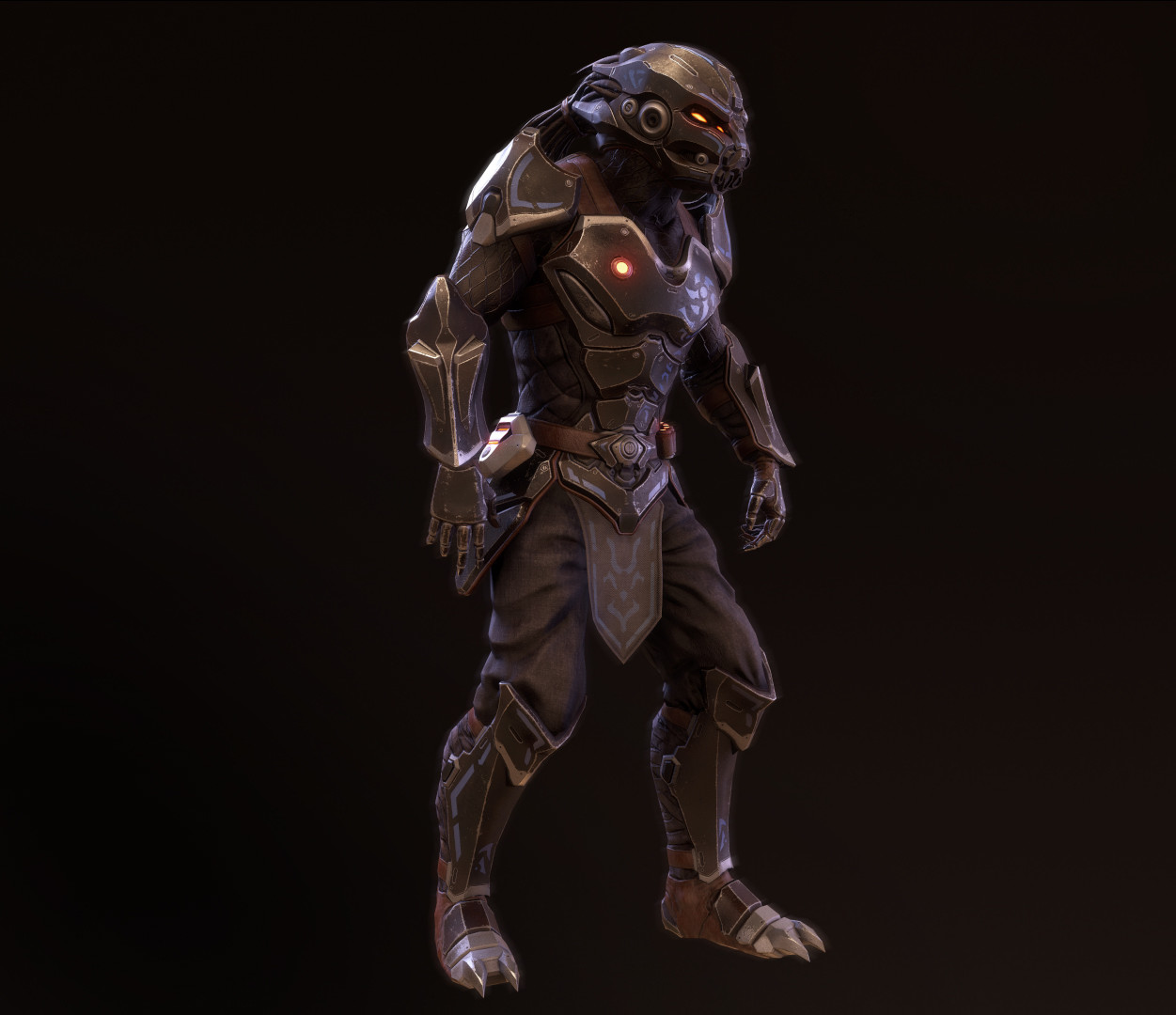The image portrays a computer-generated creature, likely from a video game or movie, set against a black backdrop. This entity is clad in intricate, brown armor that envelops its entire body, giving it a formidable appearance. The helmet, which has an alien-like design, covers the face completely, save for the glowing, slit-like yellowy-gold eyes. Its boots are constructed entirely of metal and feature silver spiked claws at the toes. The creature wears a meticulously detailed chest piece with a glowing light on the left breast, and a codpiece made of leather, adorned with mysterious symbols. An armband extends above its elbow, covered in ornate designs, paired with silver metal gloves. Around its waist is a belt, possibly acting as a weapon holster, adding to its readiness for combat. The ensemble creates a seamless fusion of fantasy and advanced technology, suggesting a character designed for a dark and immersive narrative.